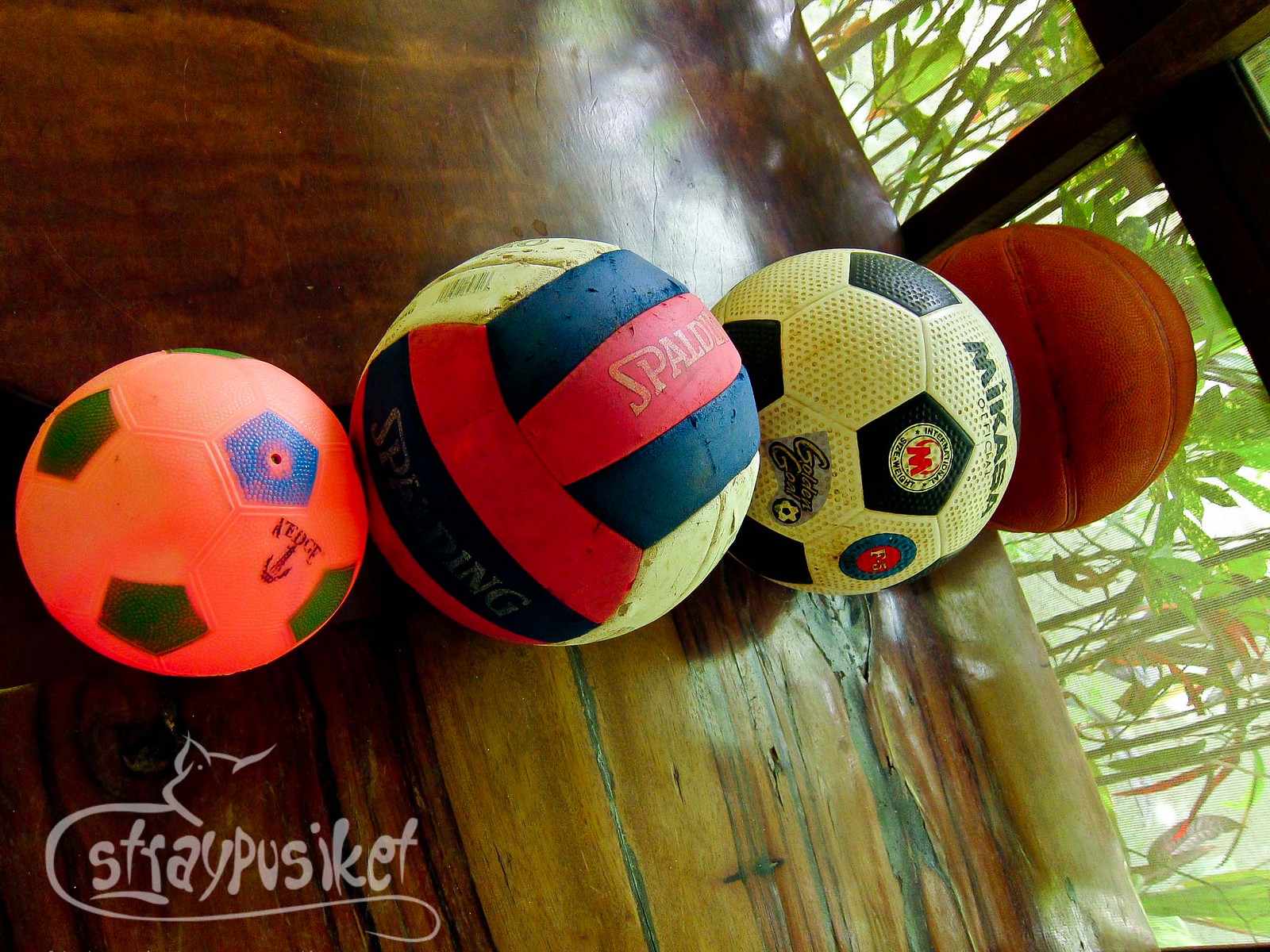This color photograph shows four sports balls—two basketballs, a volleyball, and a soccer ball—lined up in a row on a weathered yet varnished wooden deck, possibly made of teak. The image is taken at an odd, slanted angle, making the deck appear tilted, and a wire mesh fence and some greenery, possibly bamboo, are visible in the background. The first ball is a high-visibility orange soccer ball with blue and green sections. Next is a volleyball with colorful blue and red stripes and the word "Spalding" (partially visible) on it. The third is a soccer ball in off-white and black, and the last is a brown basketball, possibly unmarked. In the bottom left-hand corner, there is a stylized white cat and the words "Stray Pussycat" or "Stray Posiket." The overall scene feels dynamic due to the unusual angle of the photograph.